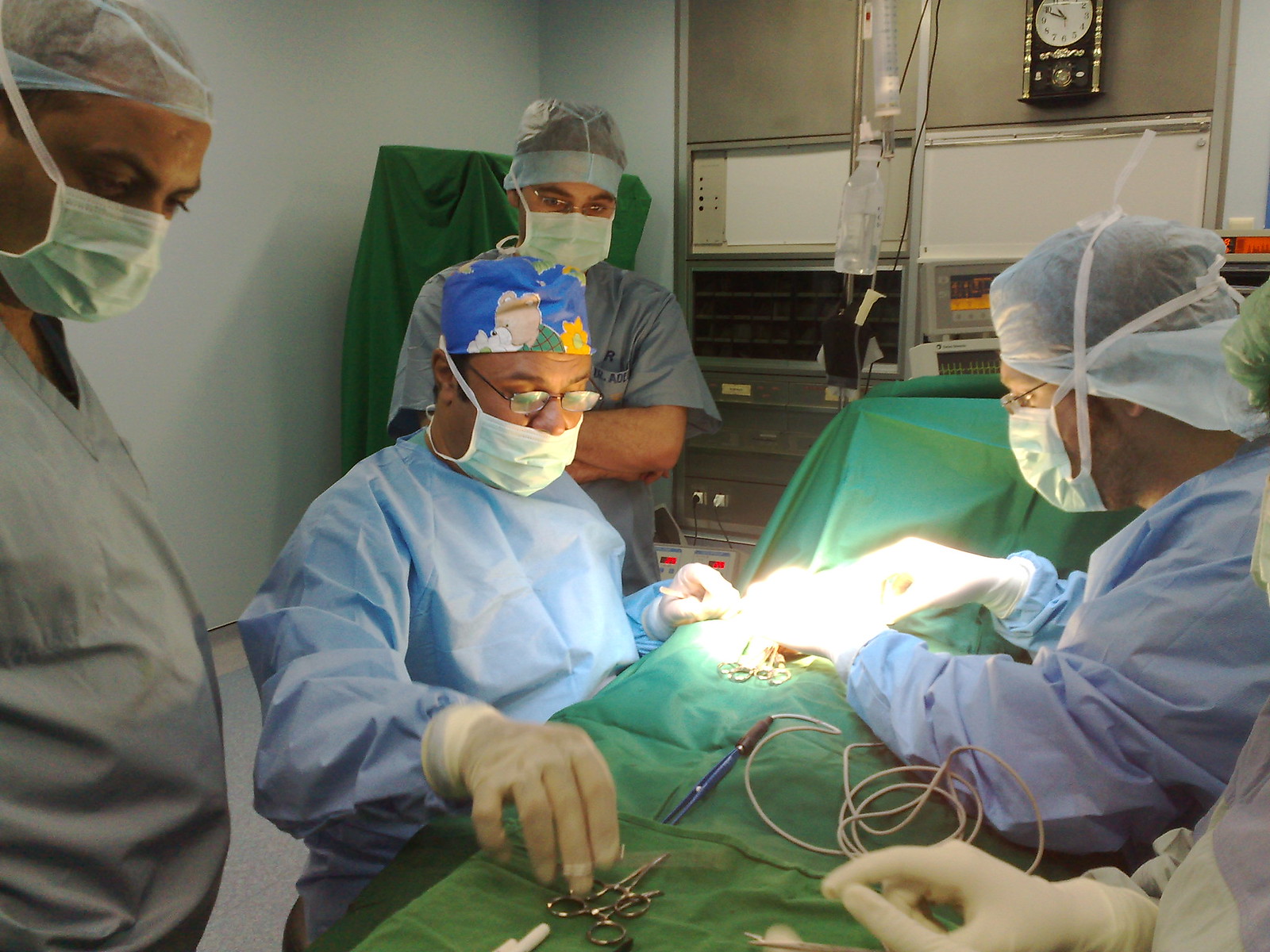This detailed full-color photograph, taken indoors in an operating room, captures a surgical team in action at 11:50 AM, as indicated by a wall clock in the background. Four medical professionals are present, all in full surgical garb, including masks, gloves, and gowns. Two individuals are positioned towards the back, with one observing the scene with folded arms. The lead surgeon, a shorter man distinguishable by his blue cap adorned with colorful designs, white mask, and blue gown, focuses intently on the procedure. Beside him, a nurse or assistant extends her arm toward the brightly lit operating area, although the intense light obscures precise details of the patient. The operating table at the center of the image is covered in green drapes, and various medical instruments, including scissors and wires, are laid out. Additional medical equipment and a variety of colors like light blue, white, brown, black, green, tan, orange, and red can be seen, further illustrating the scene’s detailed and busy atmosphere.